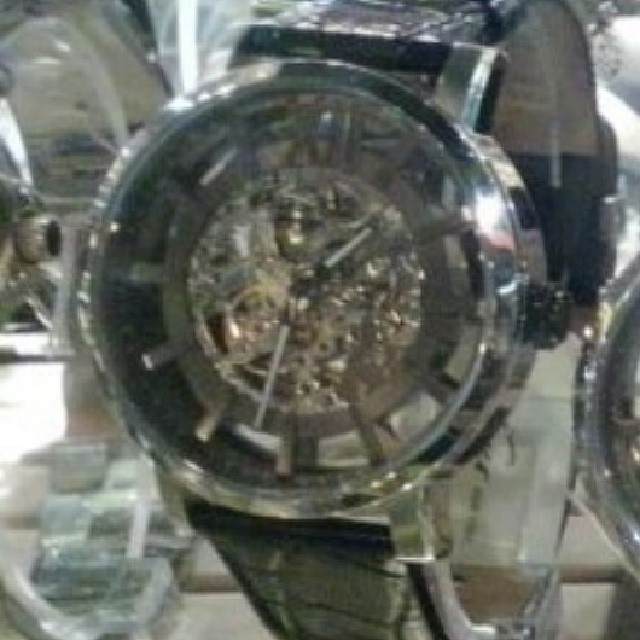This color photograph captures a blurry, very up-close shot of a fancy mechanical wristwatch. The watch is perched on a plastic stand, showcasing its elegant design. The body of the watch is predominantly silver with a sophisticated, reflective centerpiece that features visible brass and cogs, highlighting its inner workings through a clear face. The watch features Roman numerals at 12 and 2 o’clock (XII and II), while the remaining hour markers are represented by eleven silver dashes arranged around the circle.

The wristband is black on the outside and white on the inside, featuring a crocodile scale design, suggesting a mix of metallic and imitation or real crocodile skin materials. A black knob is visible on the right side of the watch face, and a partially shown wire appears on the right side of the image. The lock at the back of the wristband is also silver, adding to the overall luxurious and intricate design of this expensive-looking timepiece.